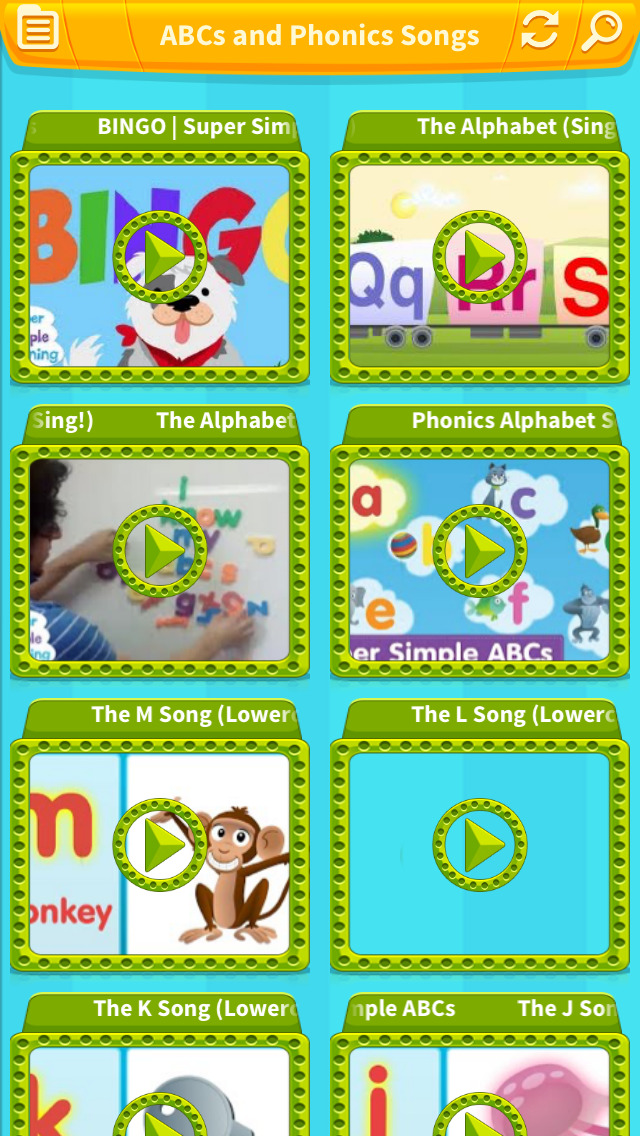The image features a brightly colored, educational interface designed for children. The primary background is a mix of orange and blue hues, adorned with playful, engaging elements. In the top left corner, a notepad icon is visible next to a refresh button and a magnifying glass, suggesting interactive search and reset functionalities.

Dominating the scene are several squares, perhaps representing different sections or categories within the application. There's a noticeable blue background and a vibrant "Bingo" section featuring a person and a dog, emphasizing the theme of the popular children's song and game.

On the right side of the image, text reads "alphabets" and "alphabet" with a green border, indicating a focus on phonics. Underneath this, there are mentions of various alphabetical songs, including "M song" (associated with a monkey) and "L song." Each song seems to be accompanied by a play button, illustrated as a ring surrounding a sideways triangle, typical of media control icons.

Further down, there's a reference to the "K song" and the broader theme of ABCs and phonics songs, highlighting the application's educational purpose. The interface includes a variety of colorful, animated characters and letters like I, K, Cs, Q, R, and S, all presented in a lively and attractive manner.

Overall, the application presents a cheerful, interactive environment rich with educational content aimed at teaching children the alphabet and phonics through engaging media.